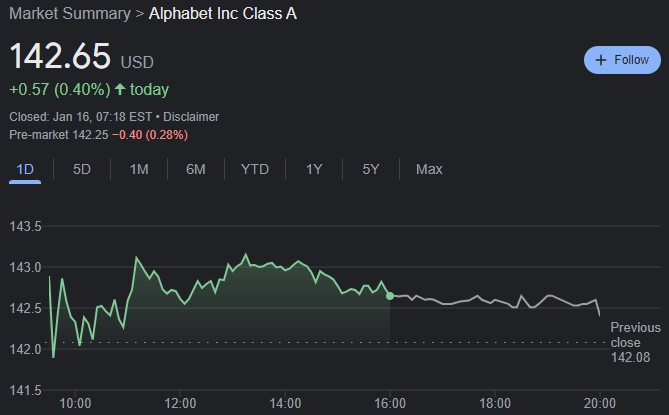A detailed snapshot of Alphabet Inc. Class A stock shows that its current price is $142.65. The chart is set to display the stock's performance over a 1-day period, among other available options including 5 days, 1 month, 6 months, year-to-date, 1 year, 5 years, and max. Key time points and prices within the selected day are noted as follows: at 10 AM, the price is approximately $142; at 12 PM, it rises to $142.50; at 2 PM, it peaks at $143; and by 4 PM, the price adjusts to $142.75. The stock has seen an increase of $0.57 or 0.40%, indicated by the green color signifying a gain. The closing time is marked as January 16th at 7:18 PM Eastern Standard Time. On the right side of the interface, there is a blue 'Follow' button with a plus sign. This appears to be a snapshot from Google's stock monitoring tool for today's performance of Alphabet Inc. Class A.